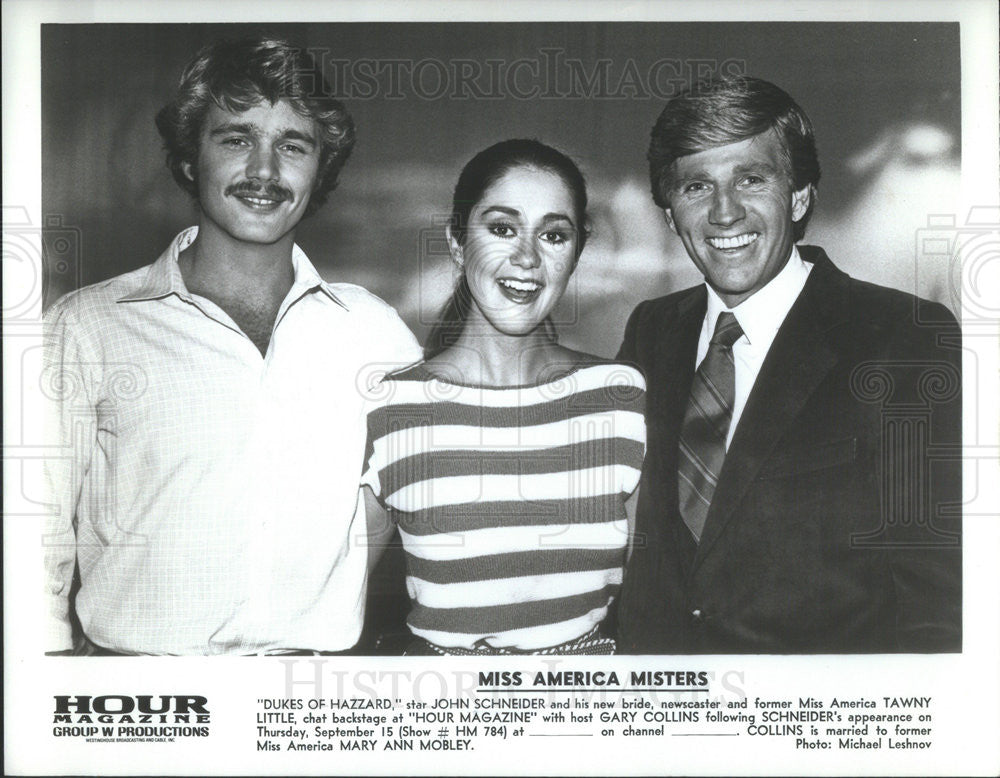This vintage black-and-white photograph, likely taken in the late 1970s, features actor John Schneider, his then-wife Tawny Little, and actor Gary Collins. Captured in a rectangular, horizontal orientation, the image showcases Schneider on the left, a young Caucasian male with curly blonde hair and a light mustache, dressed in a white button-down shirt with an open collar. His arm is around a young dark-haired woman in the center, his wife Tawny Little, a Caucasian woman appearing to be in her mid to late 20s, with dark brown hair pulled back in a ponytail, wearing a short-sleeved white striped t-shirt. To her right stands Gary Collins, a middle-aged white male with neatly combed blonde hair, clean-shaven, dressed in a white button-down shirt, a printed tie, and a black suit jacket. Below the photograph, a caption on a white background in black text reads: "Miss America Misters." It continues, "Dukes of Hazzard star John Schneider and his new bride, newscaster and former Miss America, Tawny Little, chat backstage at 'Our Magazine' with host Gary Collins, following Schneider's appearance on Thursday, September 15 (show number HM784) at blank on channel blank. Collins is married to former Miss America, Mary Ann Mobley." The lower left corner features a logo and text that reads, "Our H-O-U-R Magazine Group in Productions." Additionally, the photo is attributed to Michael Leshnov in the lower right corner. This staged moment captures the trio smiling against a gray and white backdrop, suggesting a magazine or promotional setting.